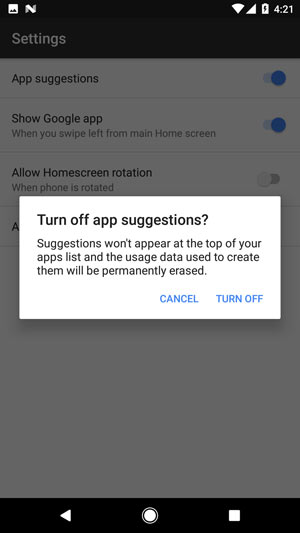Screenshot Description:

This is a detailed screenshot taken from a cell phone at 4:21 PM, evident from the time displayed on the device’s status bar at the top right corner. The status bar also indicates that the battery is fully charged at 100%. 

The primary content of the screenshot is the settings menu on an Android phone, which is visible in the background but appears grayed out due to an active pop-up window. The partial listings visible in the settings menu include options like "Show Google app" (toggled on) and "Allow home screen rotation" (toggled off).

Dominating the screen, the pop-up window is titled "Turn off app suggestions?" It informs the user that if app suggestions are turned off, no suggestions will appear at the top of the app list, and the usage data used to create these suggestions will be permanently erased. The pop-up presents two options at the bottom: "Cancel" and "Turn off."

Though the exact setting menu (whether it belongs to the Google Play Store app suggestions or general app suggestions within the Android settings) is not specified, the options presented clearly deal with the personalization and functionality of app suggestions and the Google app visibility on the device.

Overall, this screenshot captures a moment where a user is managing their device settings, particularly focusing on the toggling of app suggestions and related preferences.